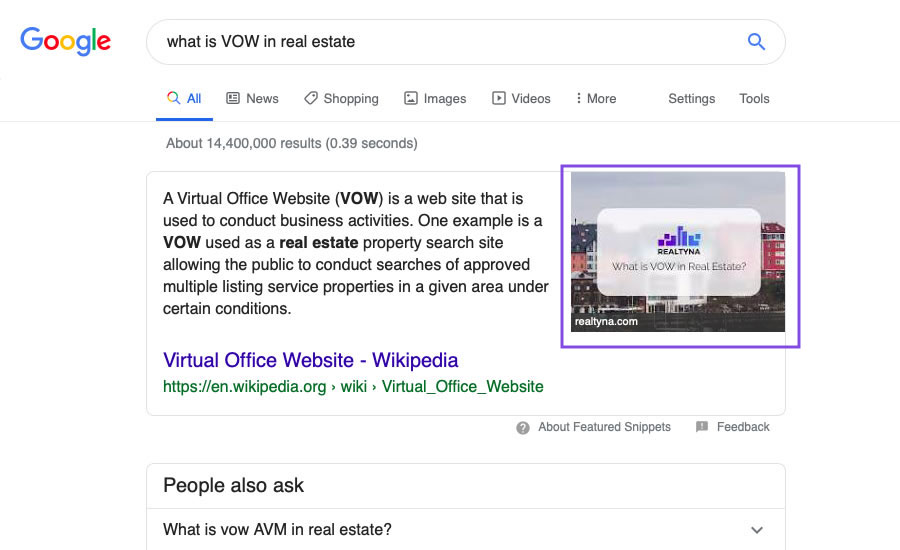The image is a screenshot of a Google search result page, prominently displaying the query "What is VOW in real estate?" The familiar Google logo in blue, red, yellow, and green colors is present at the top left corner. A search bar sits at the top of the page with a blue magnifying glass icon to its right. The selected tab, labeled "All," is highlighted in blue, featuring a colorful magnifying glass icon consistent with Google's traditional colors. Adjacent tabs include "News," "Shopping," "Images," "Videos," and additional options like "More," "Settings," and "Tools."

The search results indicate that there are approximately 14,400,000 results, retrieved in 0.39 seconds. The snippet provided for the search explains that a VOW, or Virtual Office Website, is a website used for conducting business activities. It gives an example of a VOW being used for real estate property searches, permitting the public to search for properties listed in multiple listing services (MLS) within certain conditions.

Additionally, the search results include a graphic related to real estate, possibly showing buildings and an explanatory header. The overall image offers a comprehensive look at the Google search process and the immediate information provided about the term "VOW" in the context of real estate.